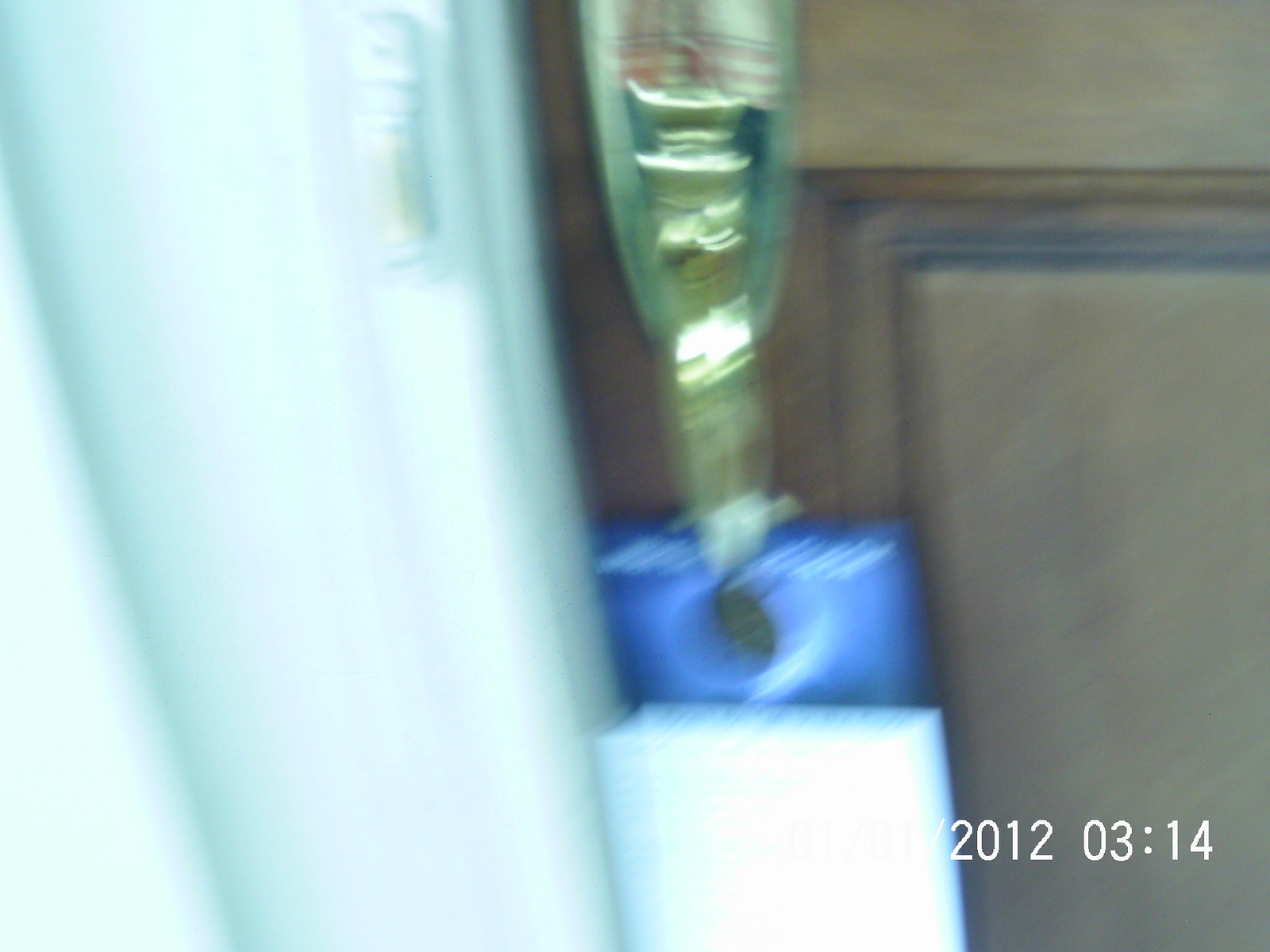This blurred photo, dated March 14, 2012, shows a scene possibly at a doorway or a cabinet handle. On the right side, a brown wooden surface with carved molding is visible, suggesting paneling or a piece of furniture. Centrally located in the image is a gold-colored object, potentially a statue or trophy, sitting on a bright blue base, which might be part of or attached to a hanging item. Below that is something white, possibly a notepad. The left third of the image features a large white object with an indistinct vertical handle, resembling the side view of a refrigerator or another piece of equipment.